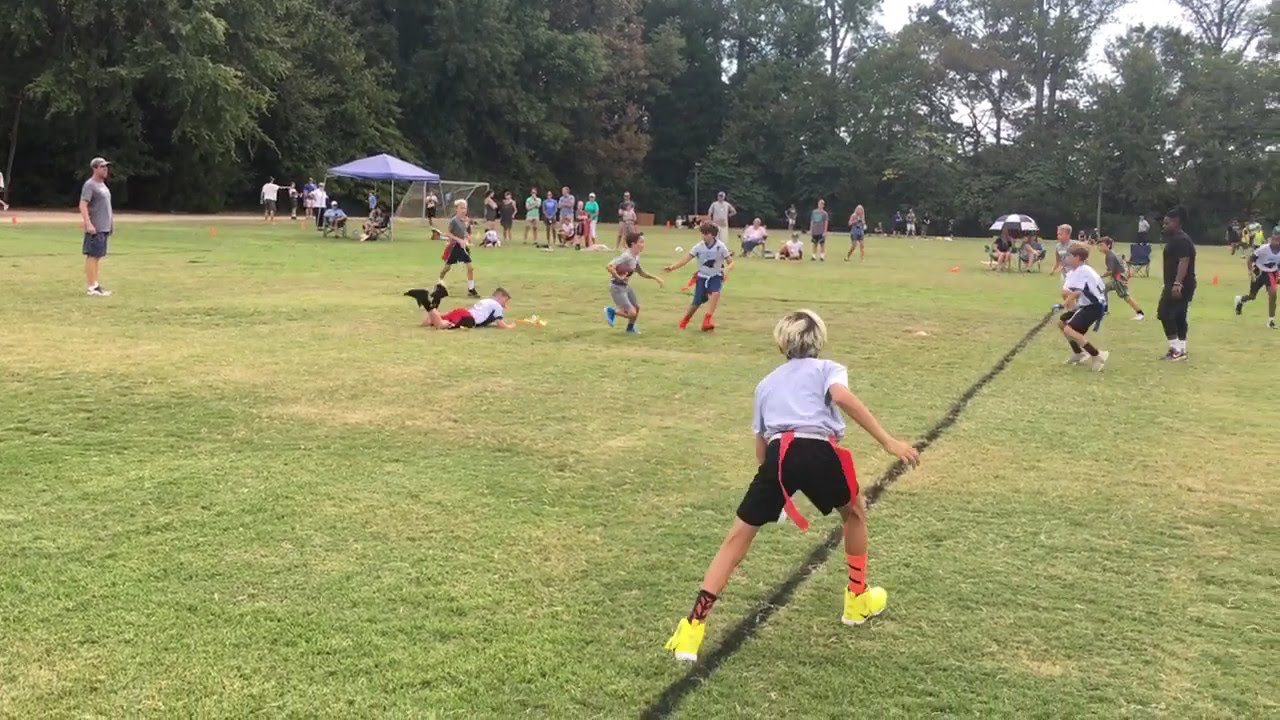In the center of a grassy field filled with patches of browning grass, a group of children is energetically engaged in a vibrant game of flag football. The gray sky looms over this bustling scene, casting a soft light over the players. In the foreground, a blonde boy wearing a gray t-shirt, black shorts, and yellow sneakers is prominently displayed, with a flag attached to his waist. Above him, several children are actively participating in the game; one boy, also in gray with blue sneakers, is clutching the football as he sprints forward. He is being closely chased by another boy who wears red sneakers, black shorts, and a gray t-shirt. Nearby, a child dressed identically to the boy in the foreground has just taken a tumble, while yet another similarly clad child stands in the background.

Further into the middle ground, two or three more children are either running toward or awaiting the boy with the football, their eyes fixed on the action. A clearly marked goal line cuts vertically through the picture from the bottom to the top, emphasizing the intensity of the game.

Spectators, likely numbering around 20 and identified as the children's parents, are arrayed along the far background, some seated in lawn chairs, suggesting a picnic-like atmosphere. Among them is a black referee dressed entirely in black, a clear figure of authority in the game. The backdrop is punctuated by a gazebo or gabled roof structure, adding a quaint, community feel to this lively scene. Beyond this, a line of trees marks the edge of the field, framing the entire tableau of youth and exuberance on an active, overcast day.